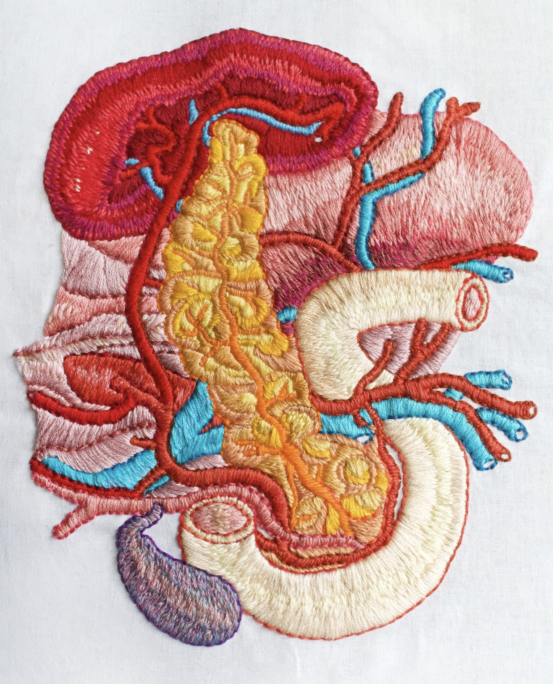The image depicts an intricate piece of handcrafted embroidery that artistically represents the inner workings of a human body. The detailed stitching showcases prominent organs like the heart, liver, and possibly the kidneys, all connected by a network of red, blue, and pink veins. At the top of the artwork, there is a shape resembling either a kidney or liver, which is linked to vibrant blue and red veins. Running down the center is a tall, slender, curved yellow and orange mass, with a large white tube snaking around its base. This elaborate creation includes a noticeable purple sac at the bottom left and varying shades of red, yellow, white, brown, beige, and pink throughout. The complexity of the colors and the meticulous nature of the embroidery make it a striking representation of human anatomy, blending artistic interpretation with detailed craftsmanship.